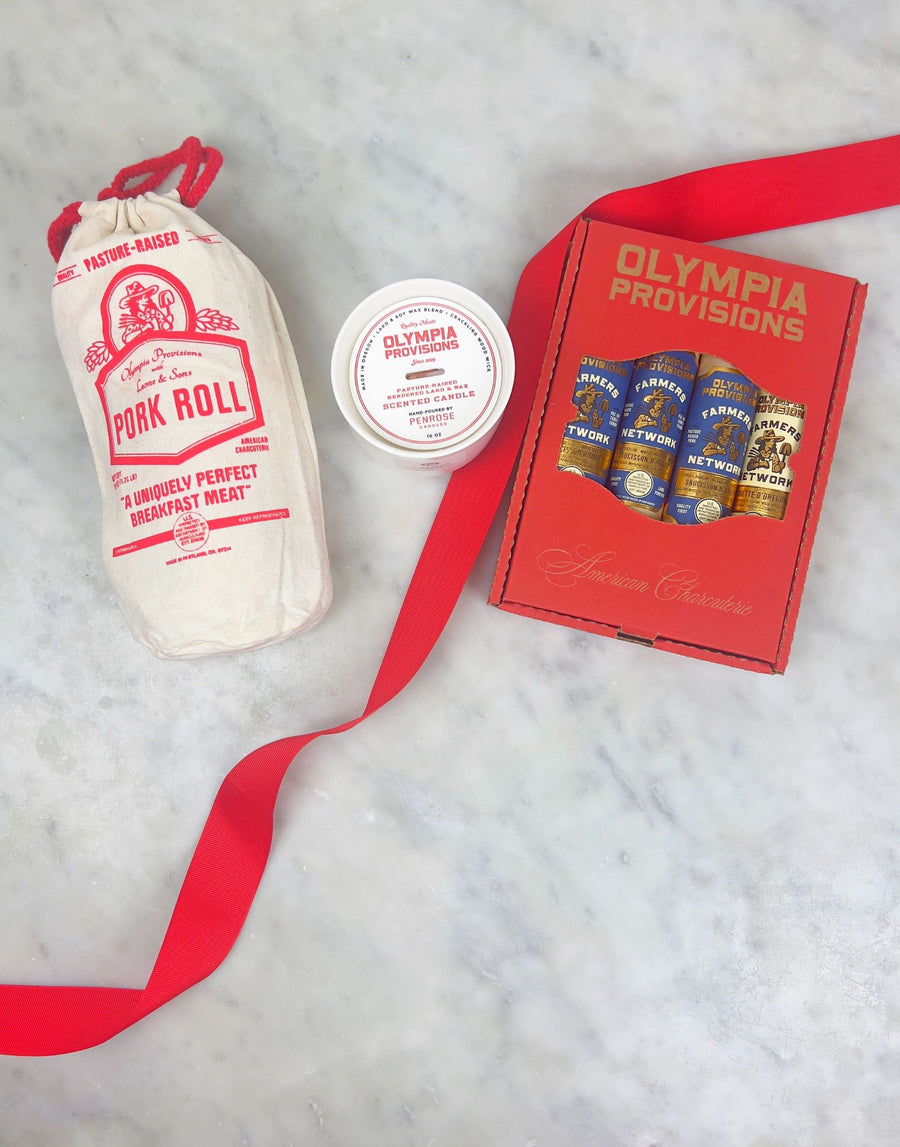The photograph features an elegantly arranged display of gourmet products on a white marble table, suggesting a Christmas gift set. Dominating the right side is a striking red box with gold lettering that reads "Olympia Provisions," showcasing clear windows revealing its contents labeled as "Farmer's Network." The items inside appear to be small, round containers or potentially gourmet sausages. To the left of the box, a vivid red ribbon diagonally crosses the table from bottom left to top right, accentuating the festive presentation. Nestled on this ribbon is a white plastic container marked "Olympia Provisions," identified as a scented candle. Continuing leftward, a tan burlap sack with red drawstrings complements the red accents of the box and ribbon. The sack is adorned with text in red that reads "Pasture-Raised Pork Roll: A Uniquely Perfect Breakfast Meat," tying the ensemble together with a rustic charm.